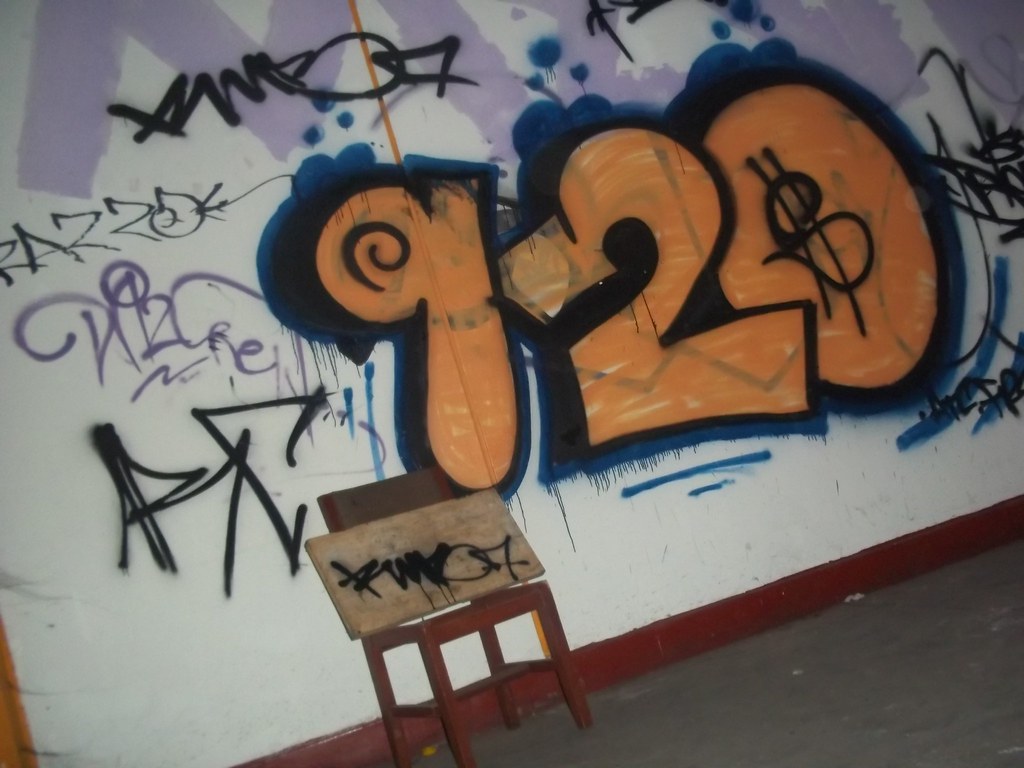The photograph depicts an indoor scene with a highly graffitied white wall featuring a prominent "920" in large, orange bubble letters, with black and dark blue outlines creating a 3D effect. The zero contains a black dollar sign. Additional graffiti, mainly in black, purple, blue, and lavender, scatters across the wall, including assorted characters and shapes, some of which resemble letters like an M or upside-down W. The wall has a dark brown or reddish baseboard at the bottom. In the foreground, a simple dark brown wooden chair holds a piece of plywood also marked with black graffiti. The floor is gray, possibly cement or asphalt, adding to an atmosphere that suggests either an abandoned house or a peculiar indoor art installation. The photo is taken at a slight angle, adding a tilt to the perspective of the wall.